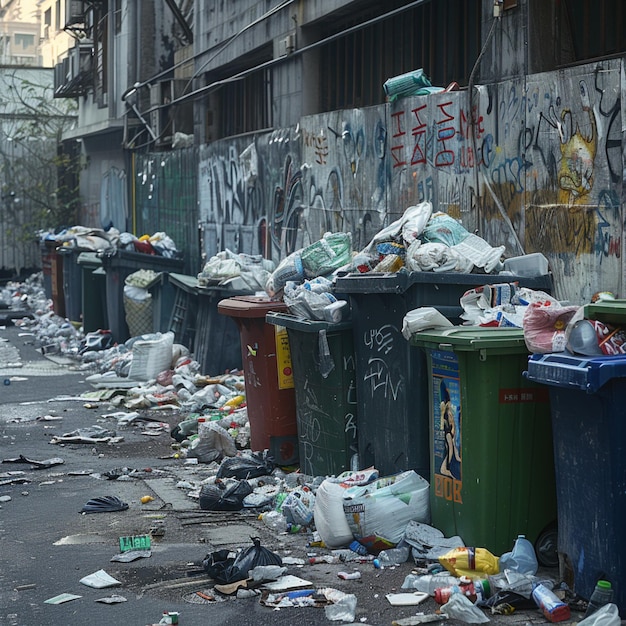The photograph captures a dreary back alley in an inner city, dominated by a line of overfilled trash bins of various muted colors—primarily blue, but with some red and green—positioned against a heavily graffitied gray wall. The wall, constructed from wood and metal fences, features vibrant spray-painted graffiti in multiple colors. A cascade of garbage, composed mainly of bottles and plastic bags, spills out from the trash bins and covers almost the entire street, obscuring the dark gray cement floor. The scene exudes a sense of neglect, further accentuated by the cloudy weather overhead. In the background, apartment buildings with visible AC units and a solitary tree peek through, adding a touch of urban residential life to the otherwise bleak, cluttered alley. The image paints a raw picture of poverty and municipal neglect, suggesting that local refuse collection services have been absent for some time.